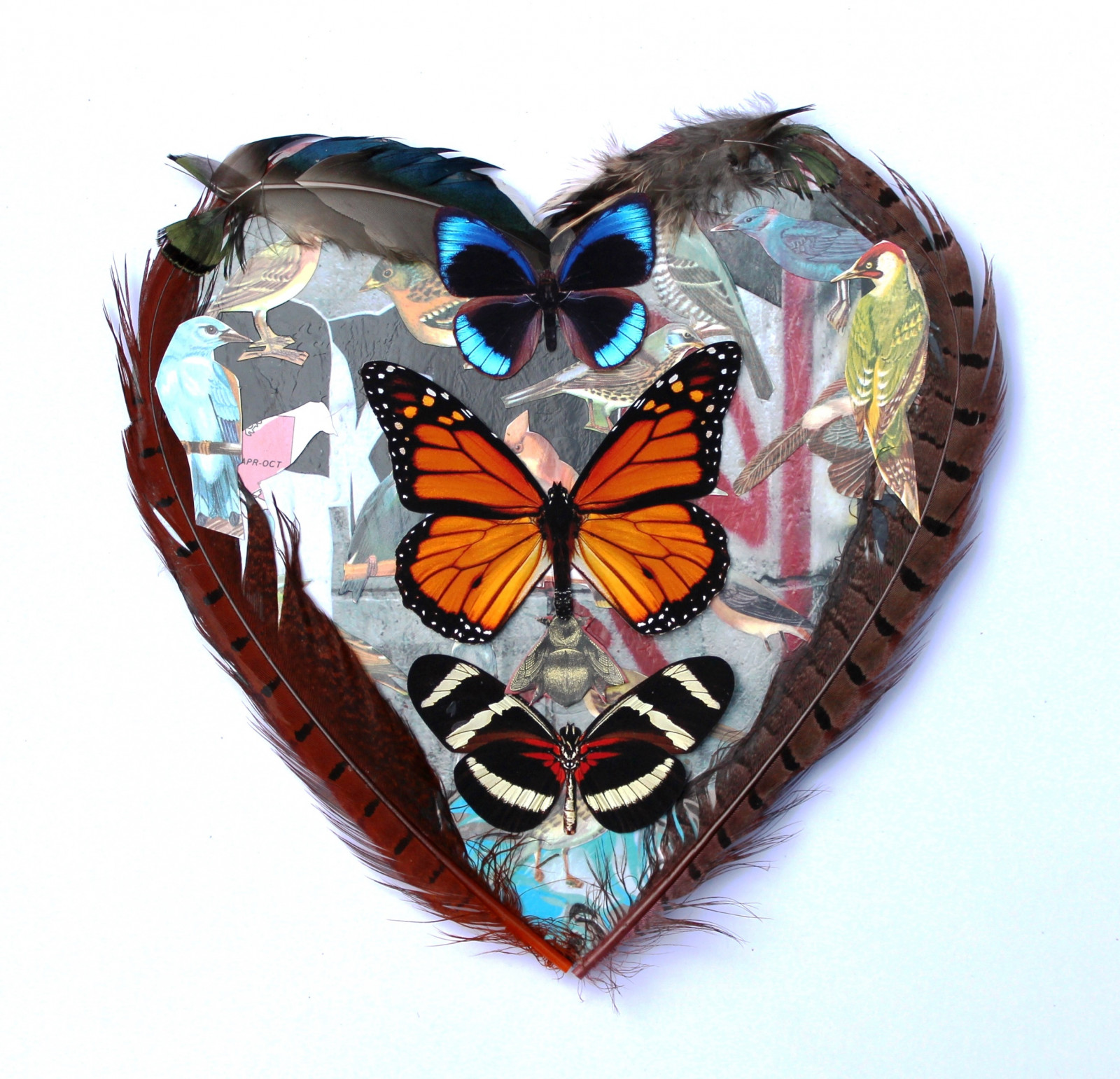This detailed artistic rendering features a heart shape intricately bordered with a variety of bird feathers, highlighting a unique blend of colors and textures. The feathers include a red feather with black grill-like marks on the left, a gray feather with iridescent blue-green accents at the top left, a fur-like gray feather at the top right, and a rust-brown feather with black markings on the right. Within the heart, against a white background, is a collage-like interior showcasing a pastiche of colors and patterns. There are cut-out images of birds, including green, blue, and orange birds, resembling pictures from a bird identification book. Down the spine of the heart, three distinct butterflies are prominently displayed. The smallest, at the top, is black with iridescent blue-green tips on its wings. The middle and largest butterfly is a classic monarch, characterized by its predominantly orange wings with black and white polka-dotted edges. The bottom butterfly features a unique pattern with a white body, transitioning into black wings adorned with red and white stripes. The heart's intricate design is neither strictly a painting nor a drawing but straddles the line between the two, creating a compelling and multi-layered visual experience.